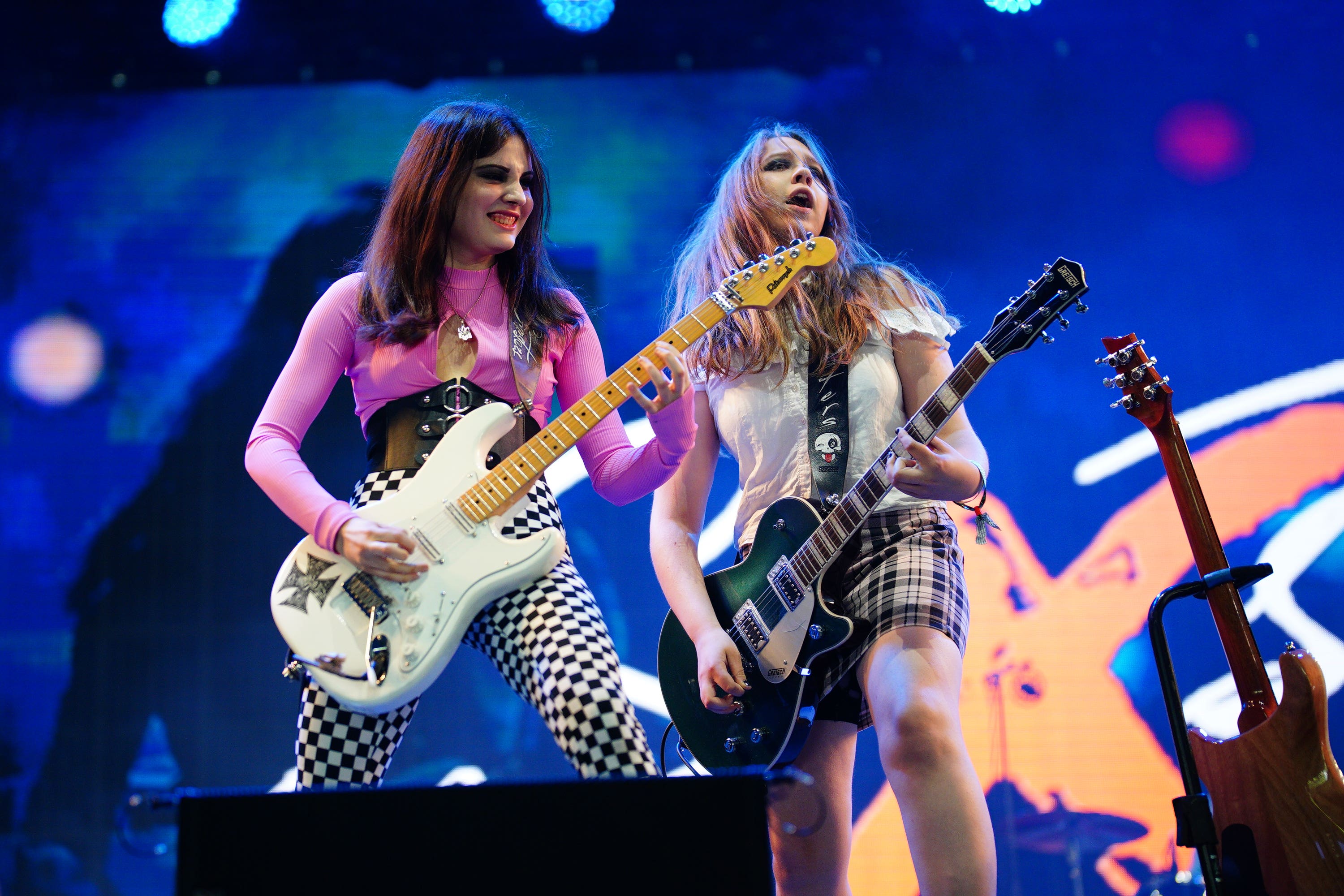This is a detailed photograph of two young teenage girls on a stage, both playing electric guitars. The girl on the left has brunette hair and is dressed in a pink long-sleeved top with a cutout on the chest, black zebra-striped pants with checkered patterns, and a wide black leather belt with silver accents. She is playing a white guitar adorned with a black cross on the upper left hand near the rear and is smiling with dark eyeliner and red lipstick.

Next to her is a blonde girl with shoulder-length hair wearing an off-shouldered white peasant-style short-sleeved top and a plaid skirt. She is playing a green guitar, with her mouth slightly open, likely singing. 

The background of the stage is deep blue with various colorful graphics including yellow, pink, light pink, and white shapes, such as an orange X and a white squiggly line. Spotlights illuminate the performers from above while a monitor is visible at the bottom of the screen, used for sound monitoring. To the right of the blonde girl, there is a light brown guitar placed on a stand. The audience is looking up at the scene, witnessing a lively rock performance.